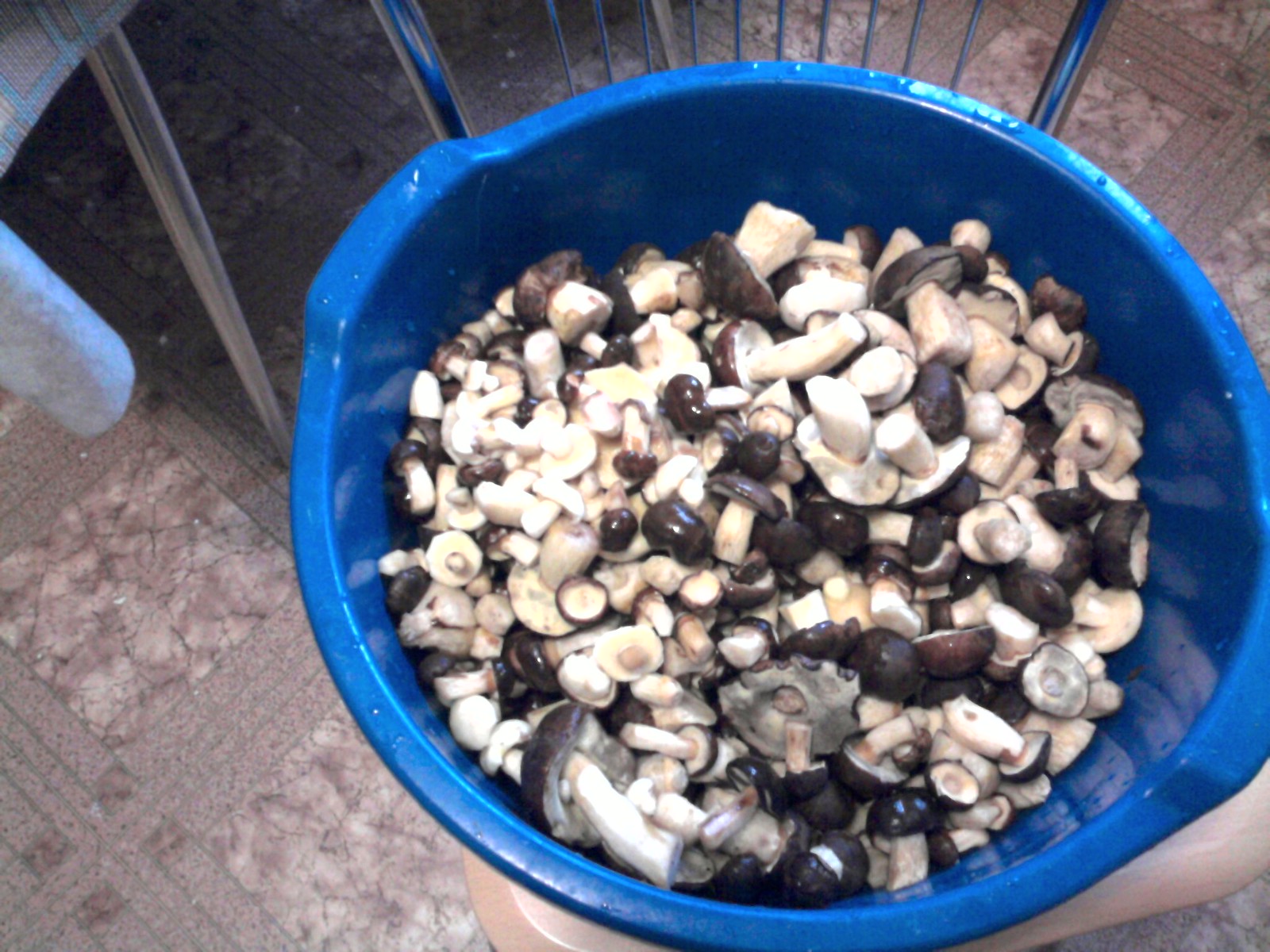This photograph captures a top-down view of a bright blue plastic bucket filled with mushrooms of various shapes and sizes, some appearing significantly larger than others. The mushrooms, with their light white stems and caps in various shades of brown, are haphazardly arranged, some showing their dark brown tops while others reveal their white filaments underneath the caps. The bucket dominates the image and appears to be resting on a chair with a beige or wood grain seat and a backrest made of chrome cylinders. Surrounding the chair and bucket is a checkered tile floor with a darker brown and pink hue pattern. In the upper left corner, part of another chair can be seen, along with a piece of fabric that might be a tablecloth, featuring a blue and brown print.